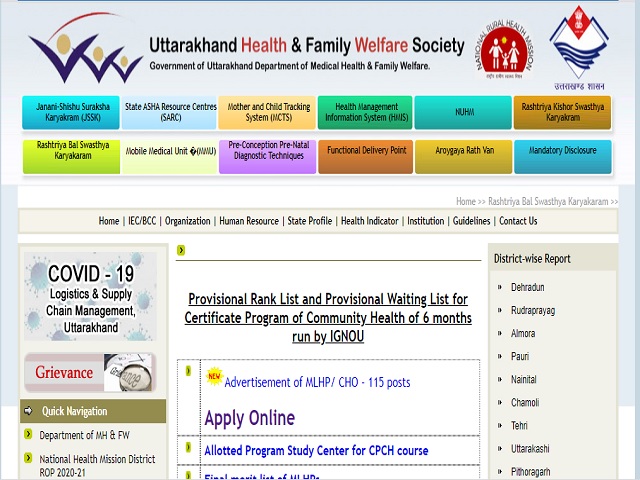The image showcases a screenshot of a webpage from the Government of Uttarakhand Department of Medical Health and Family Welfare. At the top of the page, the header reads, "Uttarakhand Health and Family Wellness Society" and "Government of Uttarakhand, Department of Medical Health and Family Welfare."

Below the header, the page is divided into sections with clickable rectangular buttons spread across two rows:

**First Row:**
1. A teal rectangle labeled "Jani Shishu Suraksha Karayakram (JSSK)"
2. A light blue rectangle labeled "State ASHA Resource Centers (SARC)"
3. A light orange rectangle labeled "Mother and Child Tracking System"
4. A green rectangle labeled "Health Management Information System"
5. A teal rectangle labeled "National Urban Health Mission (NUHM)"
6. A dark orange rectangle labeled "Rashtriya Kishor Swasthya Karyakram (RKSK)"

**Second Row:**
1. **Additional colorful rectangle buttons with various other medical and healthcare-related labels, not fully visible in the initial screenshot.**

Below these buttons, the webpage continues with more sections, lists, and detailed information related to health and family welfare programs offered by the department.